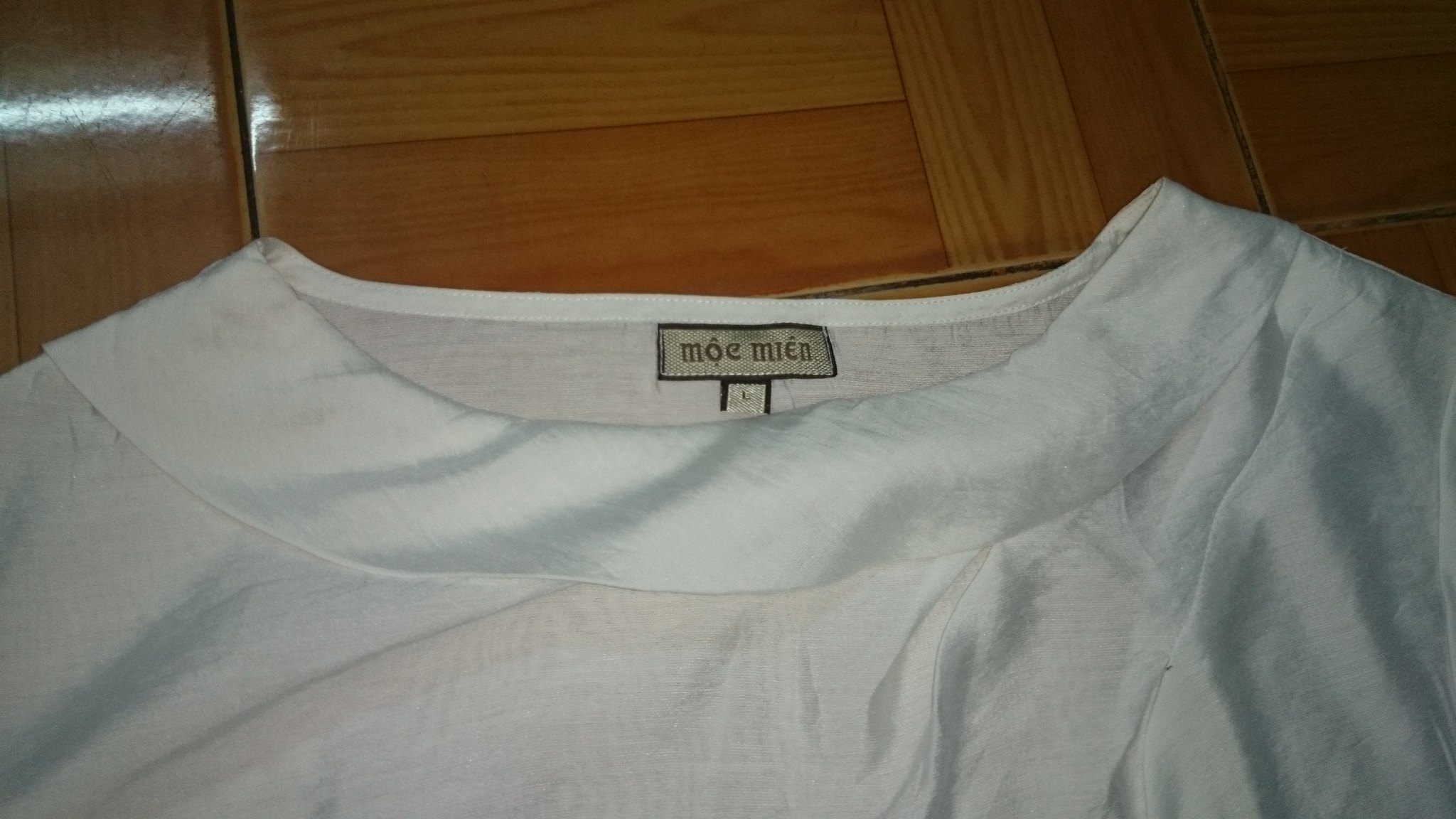This image depicts the top portion of a white t-shirt laid out on a floor of pale pine-colored parquet flooring, identifiable by the visible lines between the wooden slats that alternate between horizontal and vertical placements. The t-shirt is slightly wrinkled and features a round, flat collar that swoops slightly, resembling the style of a woman's shirt. Prominently displayed at the t-shirt's neckline is an outlined black tag labeled "Moe Miên," with inflections over the "O" and "E," and written in lowercase. Below this tag, there is a smaller square tag indicating the shirt size as large.